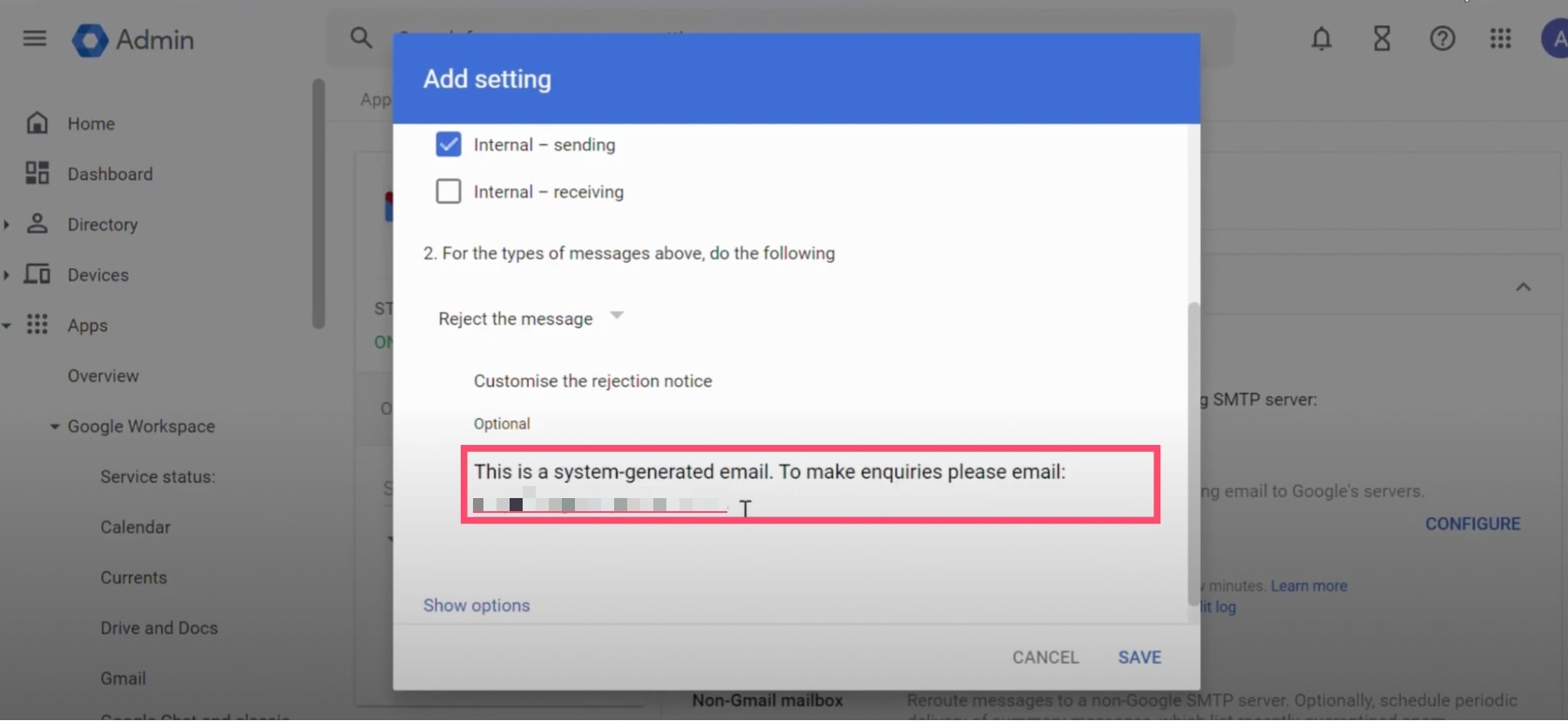The image displays an administrative dashboard interface. 

In the top left corner, the word "Admin" is prominently featured twice. Adjacent to this, a search bar is visible. On the top right, a series of icons are arranged in sequence: a bell, an hourglass, a circle with a question mark, and a grid of nine dots. There's also a blue "A" icon among them. 

On the left sidebar, there is a stacked list of menu items, which includes:
- Home
- Dashboard
- Directory
- Devices
- Apps
- Overview
- Google Workspace
- Service Status
- Calendar
- Currents
- Drive
- Docs
- Gmail

These menu items indicate various sections and tools available for the administrator.

At the center of the screen, there's a main window featured prominently. A large blue bar at the top of this window reads "Add Setting". Below it, there are segmented areas labeled as "Internal - Sending" and "Internal - Receiving." 

Within this primary window, there’s a box denoting two types of messages with options like "Reject the message" and "Customize rejection", which is optional. There's a note about this being a system-generated email, accompanied by different color highlights for various settings. A red bar highlights specific options. Buttons labeled "Show Options" and "Cancel" are clearly visible, along with a blue "Save" button.

To the right, there’s a scroll bar indicating that there are additional settings or options viewable upon scrolling. 

In the bottom right corner, highly visible settings are denoted, including text that says "SMP server" with a blue link labeled "Configure". Additionally, a note mentions the option to reroute messages to a non-Google SMTP server and to optionally schedule periodic rerouting.

This detailed caption aims to provide a comprehensive overview of the visual layout and various elements present in the administrative dashboard interface.